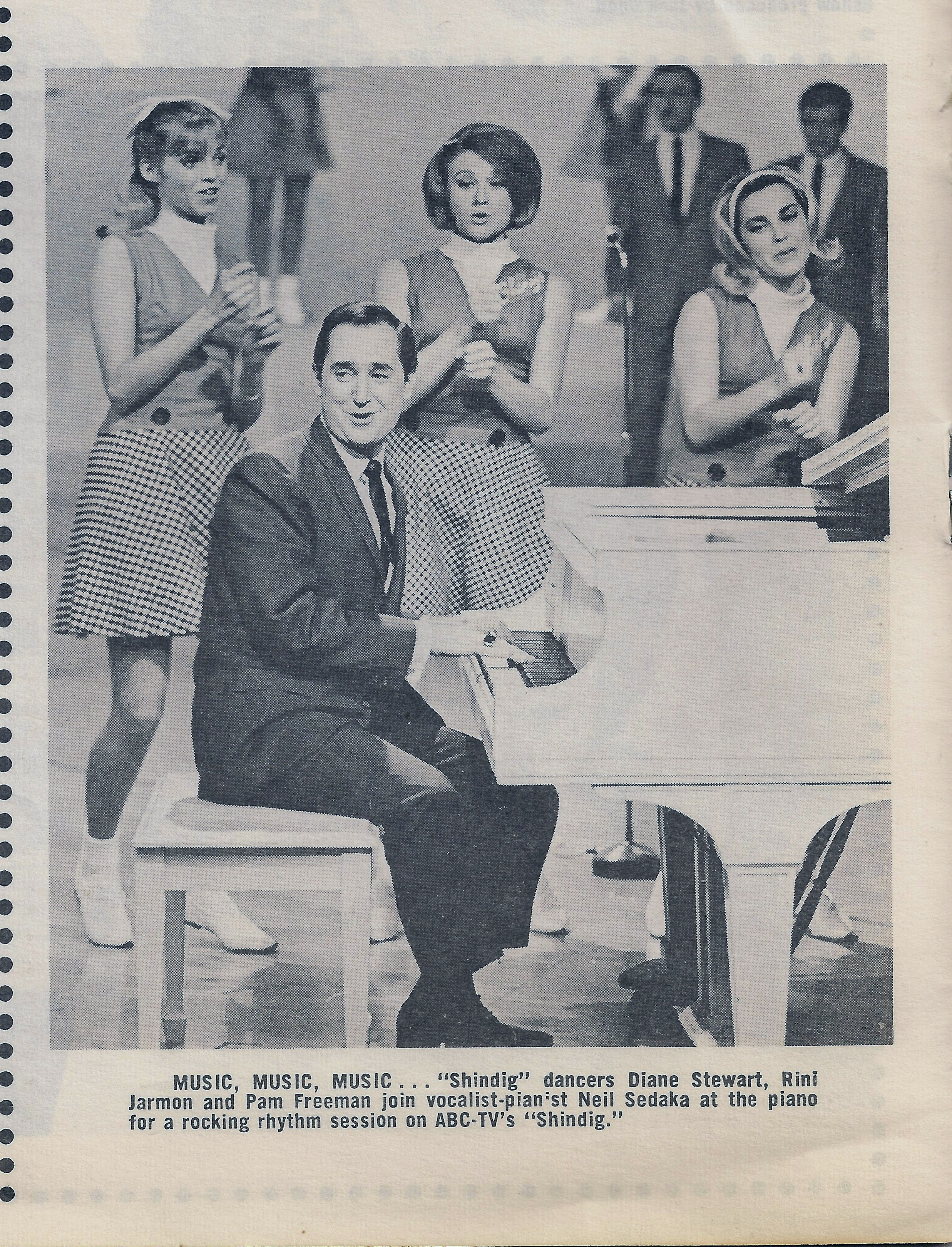This black-and-white photograph, likely from a 1960s magazine or newspaper, features a scene from ABC TV's "Shindig." The image is bordered by a light gray frame, and the caption at the bottom reads: "Music, music, music. Shindig dancers Diane Stewart, Rennie Jarman, and Pam Freeman join vocalist pianist Neil Sadaka at the piano for a rocking rhythm session on ABC TV's Shindig."

In the foreground, Neil Sedaka, dressed in a dark suit with a light-colored shirt and dark tie, is seated at a white piano, singing and playing while glancing over his shoulder to the left. Surrounding him are three young women, identifiable as Diane Stewart, Rennie Jarman, and Pam Freeman. They sport quintessential 60s attire: sleeveless vests, skirts, and white cowl-neck undershirts. The women are captured mid-dance, with bent knees and hands together, exuding joyful energy.

In the background, several men in suits with narrow ties and a couple more young women in skirts can be seen, further enriching the dynamic and lively ambiance of a typical "Shindig" session.